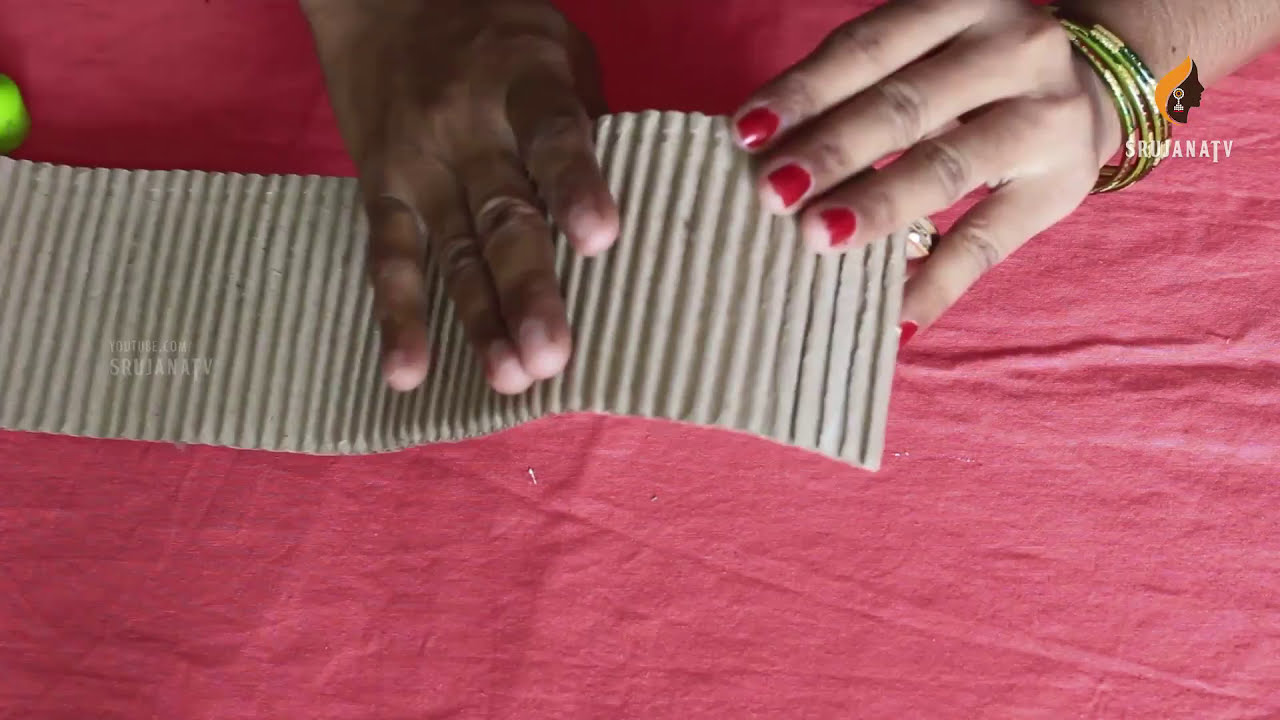The image depicts a scene centered around a pink, fabric-covered table with a slightly wrinkled texture. Lying on the table is a long, rectangular strip of corrugated cardboard, extending out of the left side of the frame. Two distinct hands are engaged in manipulating the cardboard. The right hand, with pale white skin adorned with green and gold bangle bracelets and featuring red fingernail polish, appears to be the left hand of the person on the right. In contrast, the left hand, which seems to be a right hand with darker tan or light black skin, is also holding the cardboard. Further details include a partially visible icon located in the upper right corner, featuring a gold and black design accompanied by some indistinct faded white lettering. The specific activity being performed with the cardboard remains unclear.